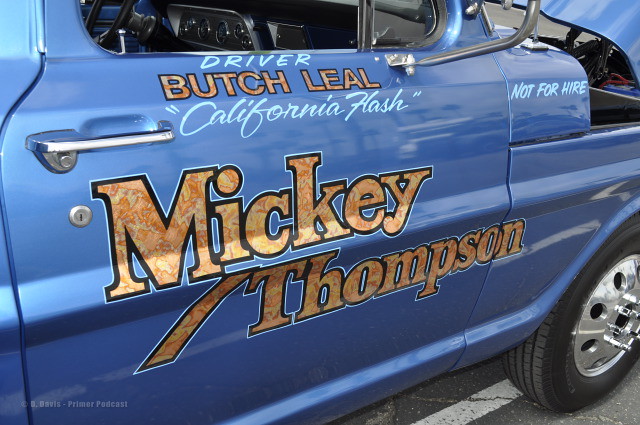The image captures a close-up of an older, metallic blue vehicle's side, focusing mainly on the door and part of the front. Prominently, the door displays the name "Mickey Thompson" in goldish-yellow lettering. Above, just below the rolled-down window, it reads "Driver" in white, followed by "Butch Leal" in matching goldish-yellow text. Beneath that, "California Flash" is inscribed in white, encapsulated within quotation marks. Adjacent to the hood, which is open, is the phrase "Not for hire." The picture reveals the black front tire with a silver rim and provides a glimpse inside the vehicle, showing the steering wheel and dashboard gauges. The car is parked on a paved road, with a white parking line visible.